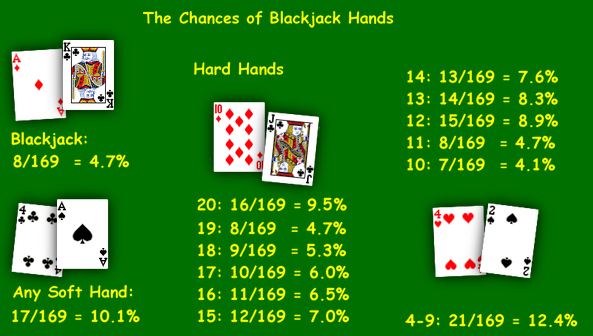This digital image has a green background with all text and numbers displayed in yellow. At the top center, the title reads "The Chances of Blackjack Hands." The image is divided into three columns: the left, middle, and right sections, each featuring pairs of playing cards with corresponding probabilities. 

In the left column, there's a depiction of the Ace of Diamonds and King of Clubs labeled "Blackjack," with a probability of 4.7%. Below this, another pair—the Four of Clubs and Ace of Hearts—is labeled "Any Soft Hand" with a probability of 10.1%. 

The middle portion lists hard hand statistics, showing pairs like a Ten and a Jack with a probability of 9.5%, and other hard hands with their respective percentages listed next to the card combinations depicted.

In the right column, statistics for lower ranking hands are shown. It includes a pair such as the Four of Hearts and Two of Spades, labeled "Four to Nine," with a probability of 12.4%. 

Overall, the image provides a comprehensive visualization of blackjack hand probabilities, combining numerical data with their corresponding card illustrations.